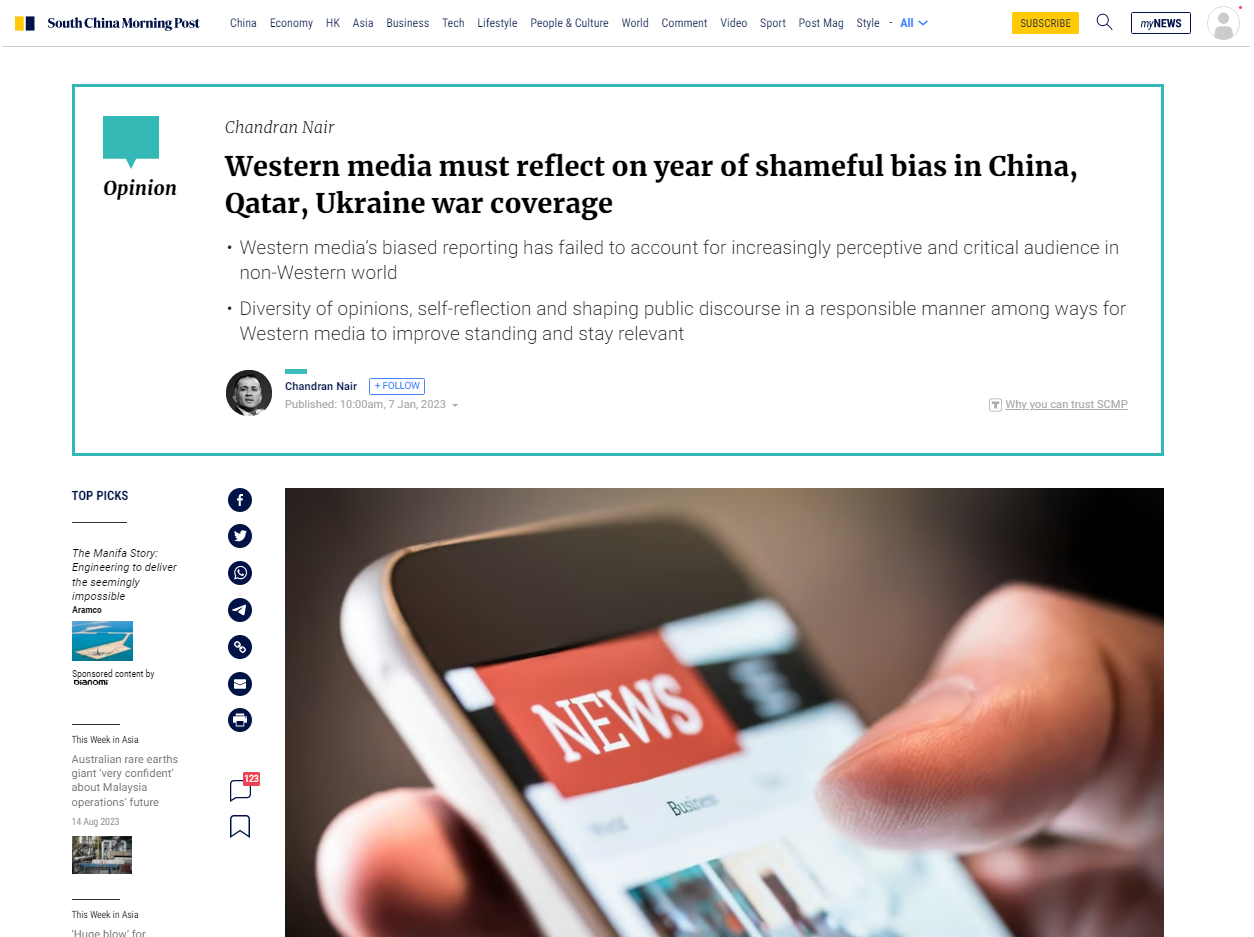This is a detailed caption for the image provided:

The image is a cropped screenshot taken from a web page rendered in a computer browser, displaying the homepage of the South China Morning Post, a newspaper-style website. Despite the browser being cropped out, the content is clear. In the top left corner, the South China Morning Post logo is prominently featured with a small yellow rectangle adjacent to a small dark blue rectangle. Running horizontally across the top, various categories are available for navigation, including Economy, Business, Lifestyle, World, and Sports. On the right side of the header, there is a yellow "Subscribe" button, a magnifying glass icon for search functionality, and a grey person icon for user account access.

Dominating the main page is a large text box with a light blue border, displaying the headline: "Western media must reflect on year of shameful bias in China, Qatar, Ukraine coverage." Directly below this headline, a significant image shows a close-up of a person's hand holding a smartphone.

On the bottom left corner of the page is a small margin containing "Top Picks," a section with brief news summaries. Adjacent to this section is a vertical line featuring multiple logos that link to external social media platforms such as Facebook, Twitter, and WhatsApp. The design and layout aim to provide an organized and user-friendly interface for readers.

Thank you for watching.